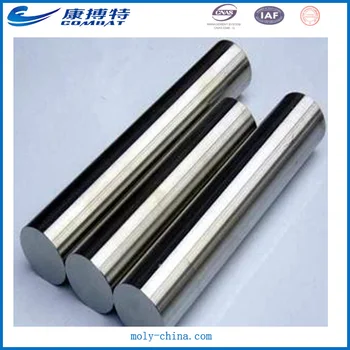This image features three polished, silver metallic rods of varying lengths, positioned at an angle of approximately 45 degrees on a white surface, likely a table. The middle rod is the shortest, flanked by a slightly longer rod on its left and an even longer rod on its right. Above these rods, the text "Combat" is displayed, accompanied by Chinese characters conveying the same word. The image includes various logos, one of which features the text "CNAS" and another that is unreadable. At the bottom of the image, the website "moly-china.com" is listed. Encircling the main image is a blue border, flanked by a red line border. A distinctive blue logo featuring a swoosh that resembles a wave appears at the top or upper left-hand corner, set against a white background, adding a cohesive visual element to the composition.